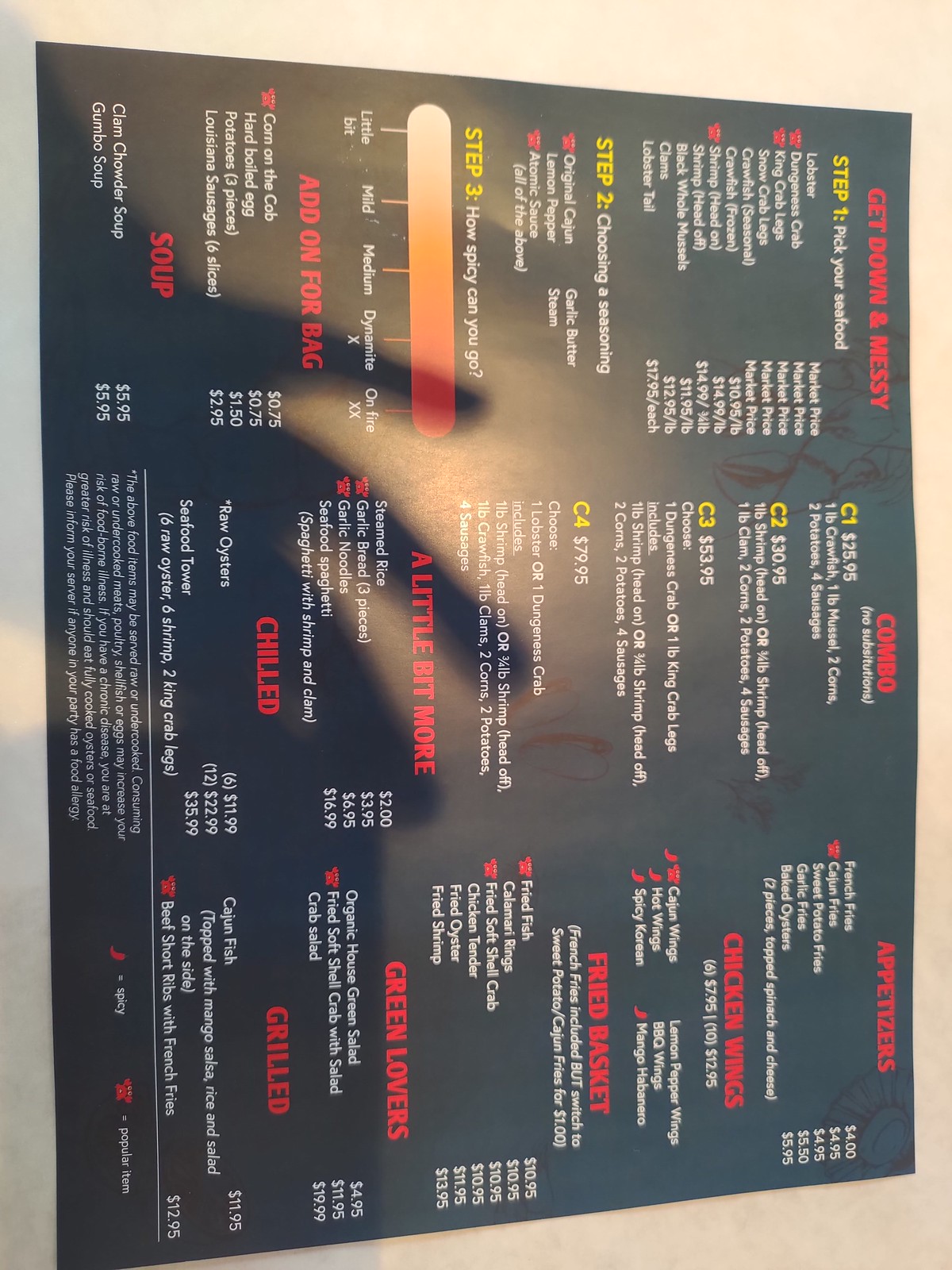The image showcases a vertically oriented menu against a light brown background. The menu itself is tilted so that the top points to the right side of the image, creating an interesting visual dynamic. The menu features a lighter black background with distinct sections highlighted in medium-colored red capital letters.

The first section header reads: "Get Down and Messy." Below this, in yellow font, it says "Step 1," followed by white font listing around ten seafood options for selection. 

Next, "Step 2" is also highlighted in yellow, instructing customers to "Choose a Seasoning," with five different seasoning options listed in white.

"Step 3," again in yellow, asks, "How Spicy Can You Go?" This section includes a spice level meter that transitions from nearly white on the left to dark red on the right, indicating increasing levels of heat.

The subsequent section, titled "Add-On For Bag," offers four options, while another section titled "Soup” provides two options for selection. The organized and colorful layout of the menu makes it easy for customers to follow the steps in customizing their meal.